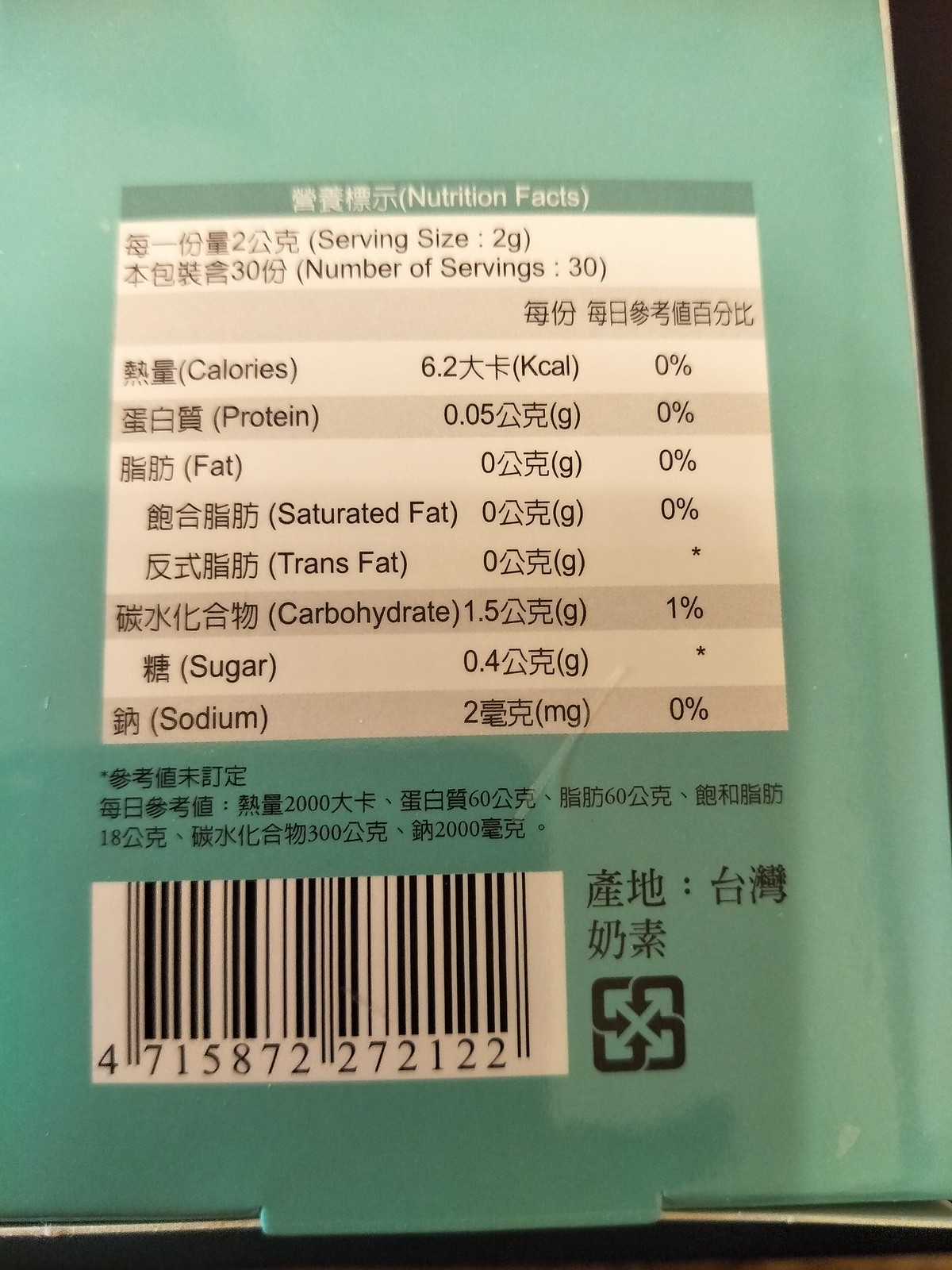This is a vertical color photograph focusing on the back portion of a product, likely a food item. The background of the product is a solid green, providing a stark contrast to the detailed content on display. Prominently featured are the nutritional facts, presented in a hybrid format with both an Asian language—possibly Korean or Japanese—and English translations. The nutritional information is organized into rows, which are highlighted with varying shades of brown for visual separation.

Below the nutritional facts, a comprehensive ingredient list is visible, though it is entirely written in an Asian language, preventing easy identification of the listed items for non-native readers. In the bottom left corner of the photograph, a barcode is present, complete with Western numerals running across its base. Adjacent to the barcode, additional Asian characters are printed, lending further authenticity and context to the product's origin and details.